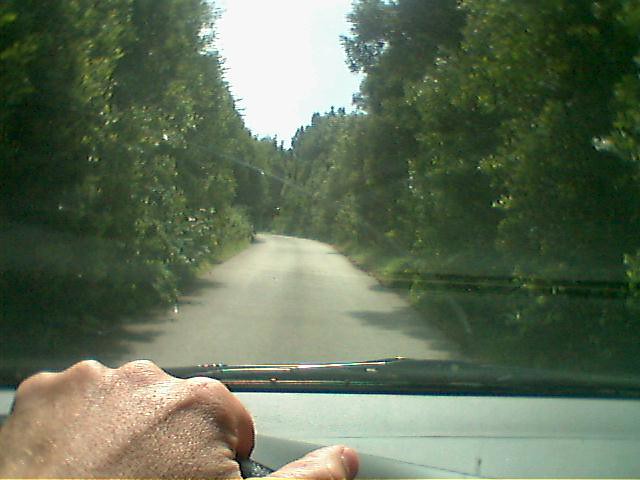In this image, we see the view from the driver's seat of a car, specifically focusing on the left hand that is gripping the top of the steering wheel. The person’s face and body are not visible, only their hand on the wheel. It's a sunny day with bright, clear skies, though there may be a few clouds. The road ahead is a narrow, grey asphalt path lined densely with leafy, green trees on both sides, casting shadows on the road. There’s no sidewalk, suggesting a quiet backcountry road. The windshield and dashboard of the car are clearly visible, with the former showing reflections and fitted with windshield wipers. The dashboard has a grey plastic appearance, and the bright sunlight even catches the driver’s hand, indicating the high visibility conditions.